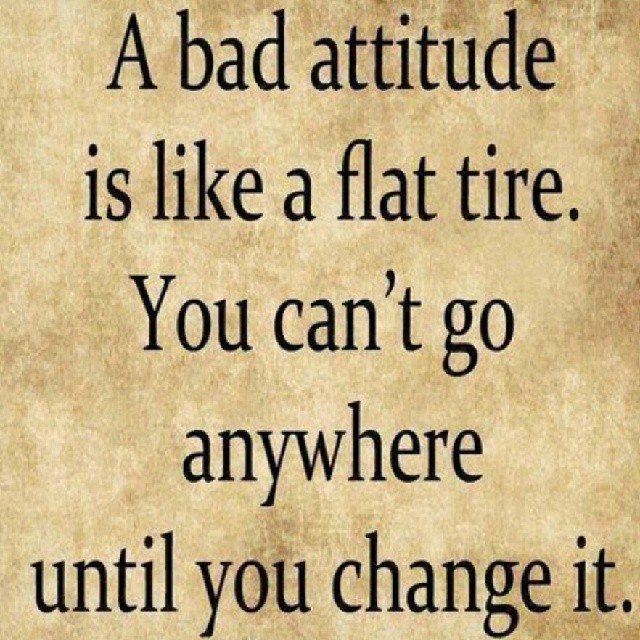The image showcases a motivational phrase in bold, black type font against a variegated light brown and white background that lends an antique-like appearance. The text is expressed in two sentences: "A bad attitude is like a flat tire. You can't go anywhere until you change it." Both sentences are properly punctuated with periods. The capital letters “A” and “Y” mark the start of each sentence. The mottled background, blending hues of light brown, tan, and white, spans the entire square, complementing the black lettering that is evenly spread from top to bottom.